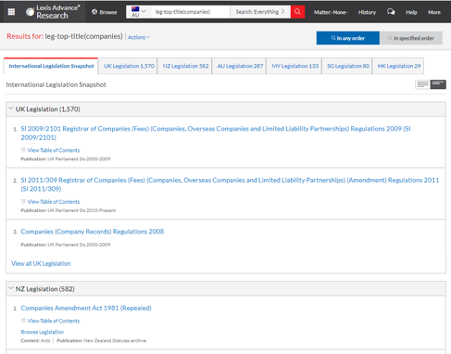The top section of the image features a black border with the text "Lewis Advanced Research" prominently displayed. To the right, there's a search box accompanied by an Australian flag and a dropdown menu. Adjacent to this, a red button is visible, and further to the right, the words "History and More" are displayed.

Beneath this section, a heading states "Results for Leg-Top-Title (Companies)". Below this, there are seven distinct tabs, each containing text in blue. The first tab on the left is currently selected and reads "International Legislation Snapshot". Under this tab, the following text is displayed:

- "UK Legislation 1.570"
- "SI 2009/2101 Register of Companies, Companies Overseers, Company, and Limited Liability Partnerships Regulation 2009".